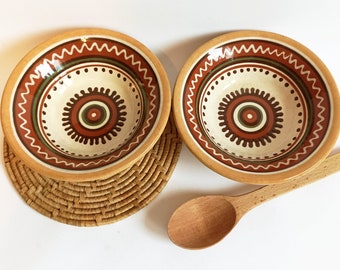The image displays a pair of shallow, identical ceramic bowls resting on a white table beneath a stark white background. The bowl on the left sits atop a light tan, circular wicker placemat, while the right-hand bowl lies directly on the table. Toward the bottom right of the frame, a large, broad-fronted wooden spoon extends with its handle pointing to the right. Both bowls exhibit intricate Native American-style designs with a light orange-brown outer edge and a darker brown rim adorned with white zigzag patterns. Inside, concentric circles alternate between colors: a thin white ring, a thin black ring, a reddish-brown band with white squiggly lines, and further inward, a dark green ring surrounding a white base featuring a central motif that resembles an eye with dark lines radiating out like eyelashes, bordered by a brown ring. The bowls cast soft shadows, suggesting that the lighting is coming from the right-hand side.